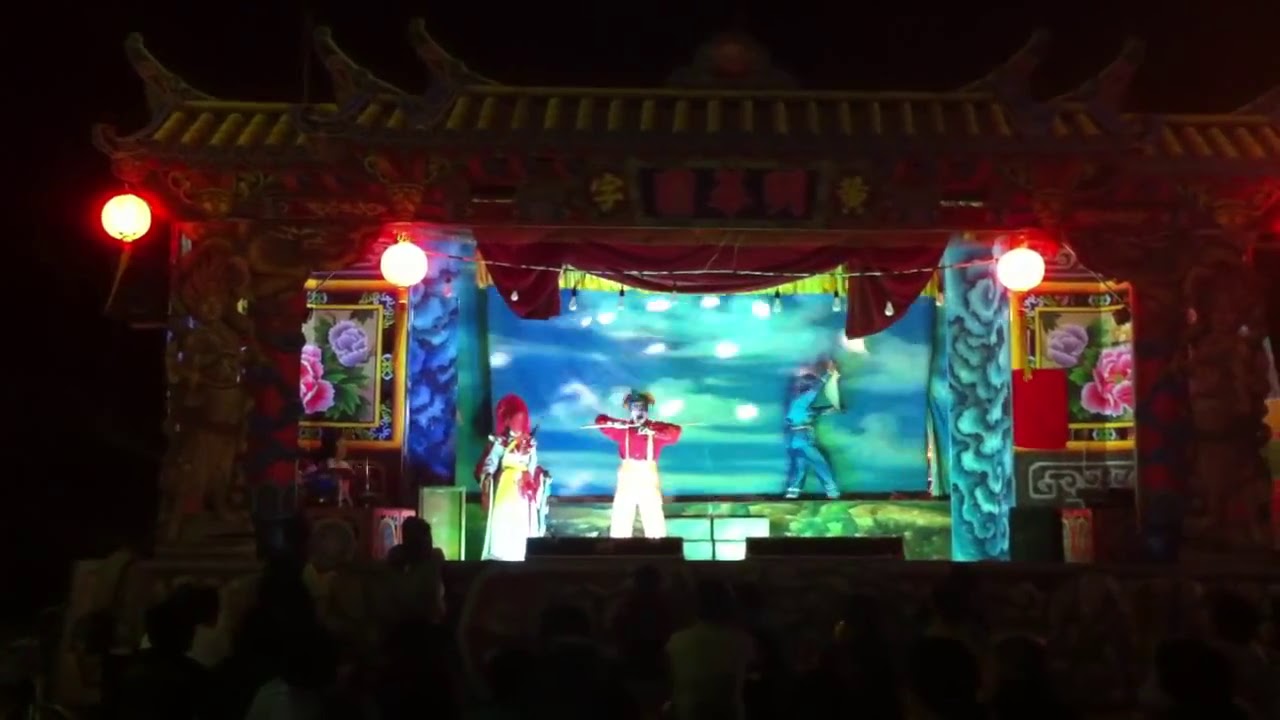The photograph captures an evocative scene from an intricately staged traditional Asian theatre production set at night. The dimly lit background suggests a theatre stage with subtle blue sky and heavy white clouds, along with a grassy area and a roadway depicted as part of the scenery. Dominating the stage are three characters adorned in vibrant costumes. 

At the center is a young woman, who commands attention with her white and yellow ceremonial dress and a distinctive red head dress. She is facing the audience, her costume amplified by a red kerchief at her waist. To her right, a man stands in white trousers and a red shirt, accented by white suspenders. His arms are bent at the elbows, with his hands positioned just under his chin and across his chest, as he gazes toward the woman. 

On the right side of the stage, another individual dressed in a bluish-gray outfit appears to be in motion, walking off-stage, disengaged from the central action. 

Embellishing the scene are vertical rectangular banners on both sides, featuring black backgrounds with paintings of pink and possibly blue or lavender roses, and Oriental writing adorning their bottoms. Two red lanterns hang from the top corners of the stage, flanking the traditional tiled roof with Chinese characters. Floral designs and varied hues of blue and green enhance the stage’s aesthetic, along with strategically placed lights that add depth to the scene. 

A barely perceptible audience sits in shadow at the bottom of the image, their heads and shoulders just visible in the darkness, creating a sense of anticipation and engagement with the dramatic tableau unfolding before them.